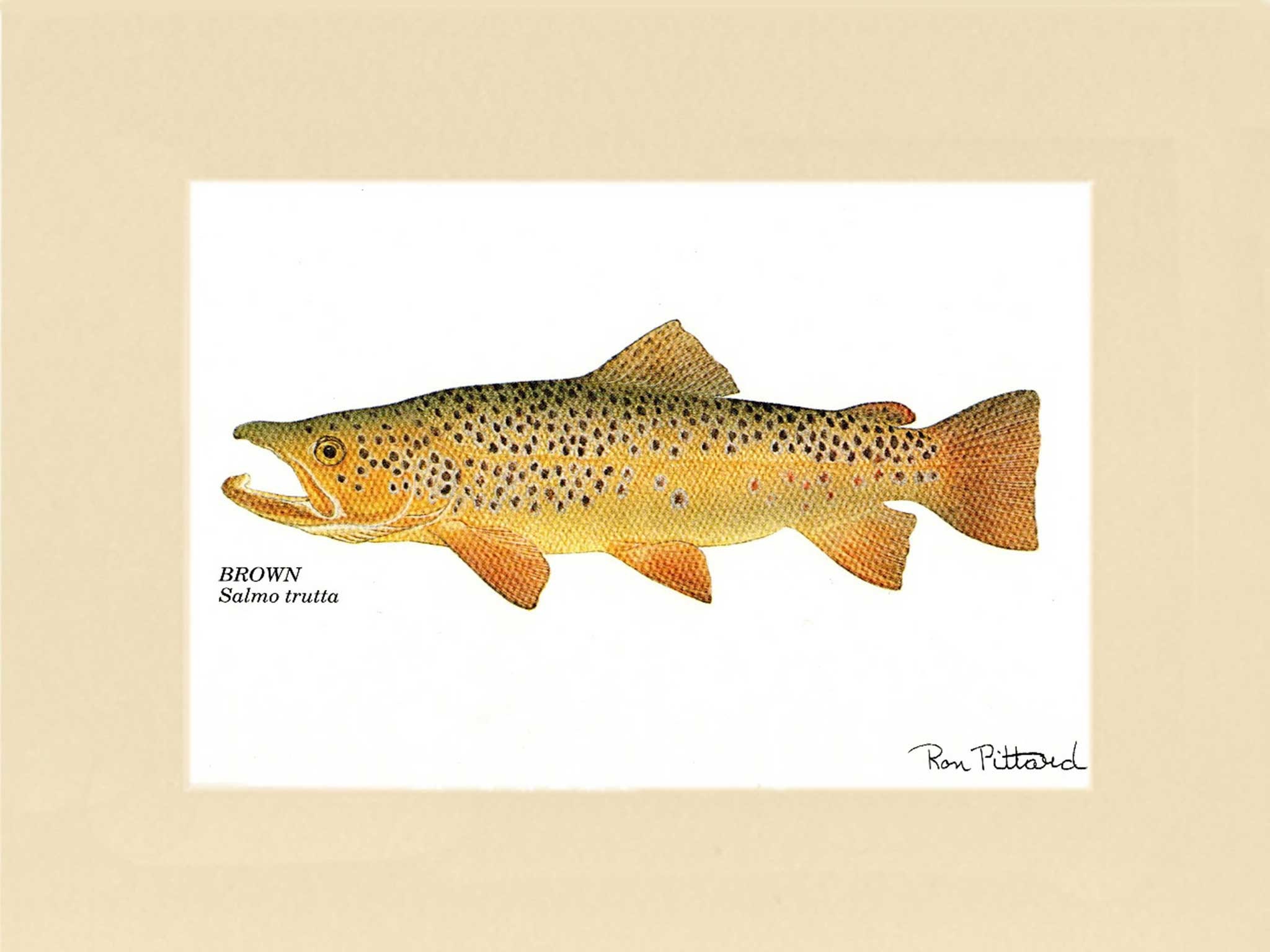This is a hand-drawn image of a fish, specifically a brown salmon, with the text "Brown Salmo Trota" in black on a white background to the left of the fish. The fish itself is depicted with intricate details: its body features a goldish-brown color on the bottom, transitioning to green on top, and is covered in distinctive black spots from its eye to its tail. The fish’s fins are orange, and it has a prominent black eye with an open mouth, giving it a lifelike appearance. The image is framed by a thick beige border, creating a classic picture frame effect, with the artist's signature, "Ron Pitard," elegantly inscribed in cursive in the bottom right-hand corner. The overall composition suggests the fish is laid flat, showcasing a side view of its complete body, including its jaw and multiple fins.